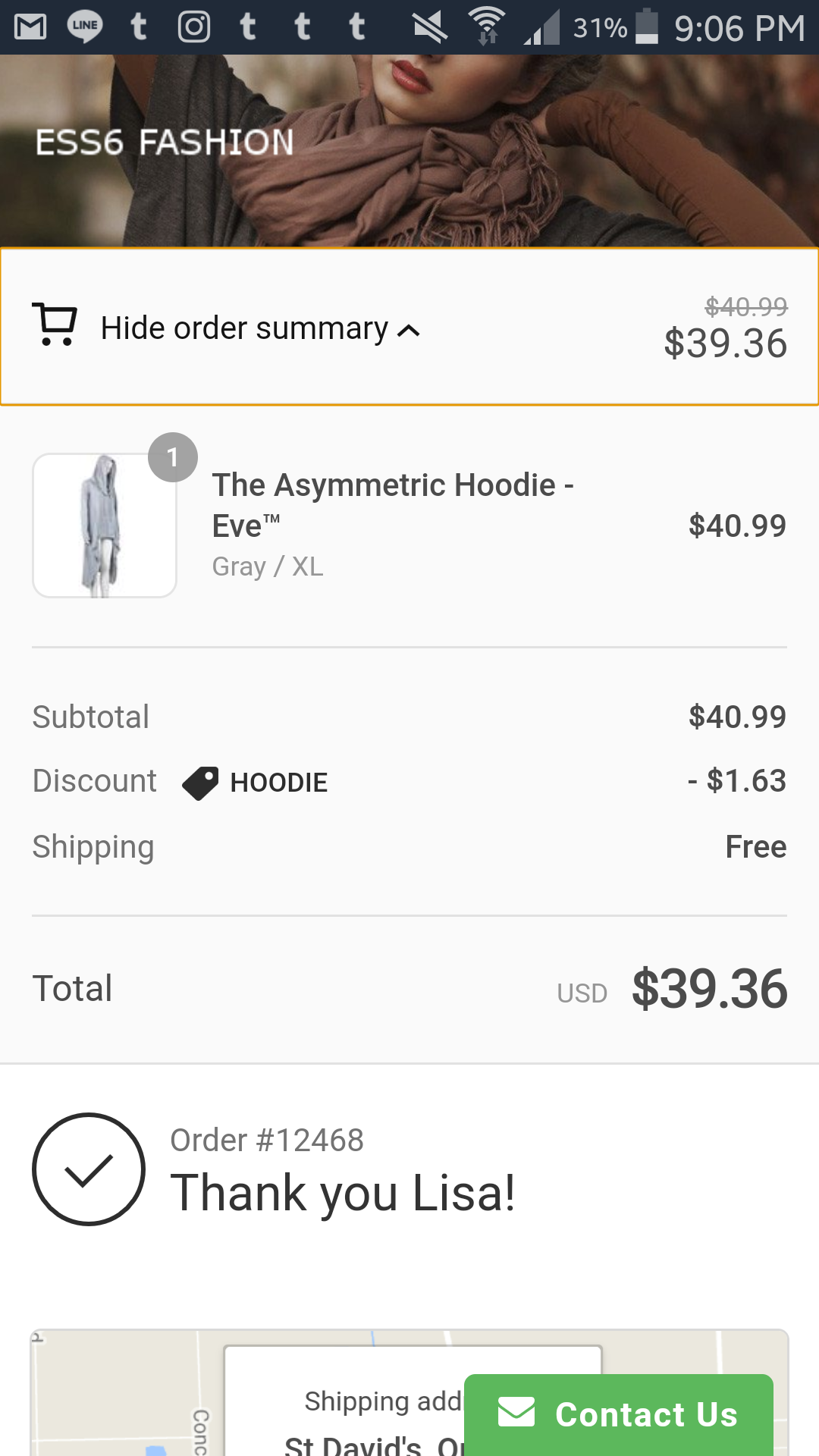The screenshot displays a smartphone interface at 9:06 PM with a 31% battery level and two out of four bars of signal strength. At the top, there are various app icons including Facebook, Instagram, and an app represented by a square with the letter 'M'. 

Below the status bar, the content reveals an e-commerce page featuring a fashion item. The header image partially shows a person's shoulders and the lower part of their face, adorned with a scarf. The caption next to this image reads "ESS6 Fashion" and "Hide Orderry Summer." 

The item listed is an "Asymmetric Hoodie" by Eve available in gray, extra large. Initially priced at $40.99, the price is marked down to $39.36. 

In the summary section, the order details are laid out: 
- Quantity: 1 
- Item: Asymmetric Hoodie by Eve, Gray, Extra Large 
- Original Price: $40.99 

A thin line separates this from the pricing summary that details:
- Subtotal: $40.99 
- Discount (hoodie): -$1.63 
- Shipping: Free 
- Total: $39.36